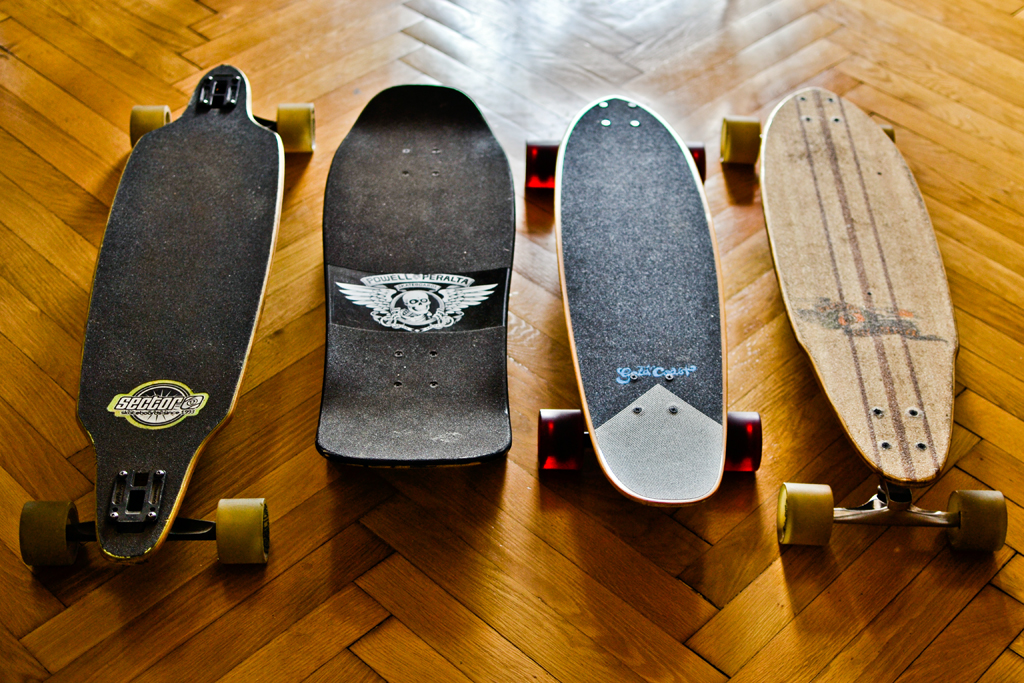In this detailed overhead photograph, we observe four distinct skateboards lined up in a row on a light brown, parquet-patterned wooden floor. Each skateboard varies in design and appearance, highlighting unique characteristics and artistic details.

From left to right:
1. The first skateboard is noticeably longer and thinner, featuring a black deck with a rough, textured grip surface. It has yellowed wheels and a circular emblem at the center, reading "SECTOR" in yellow text.
2. The second skateboard, smaller in size, is entirely black, adorned with a striking emblem of a skull with wings at its center, labeled "POWELL PERALTA." This board’s wheels are not visible.
3. Adjacent to it, the third skateboard is also black with an elongated triangular or trapezoidal design in gray on its deck. Its red, translucent wheels add a pop of color and contrast to its otherwise dark surface.
4. Lastly, the skateboard on the far right stands out with its light brown, wood-like appearance, accented by yellow wheels. The deck appears worn and features a faded black and orange design, resembling a snake.

The wooden floor beneath the skateboards has a distinct cross-hatched pattern, creating an elegant backdrop that complements the varied designs of the skateboards. The shadows beneath each skateboard suggest lighting from above, adding depth to the composition.